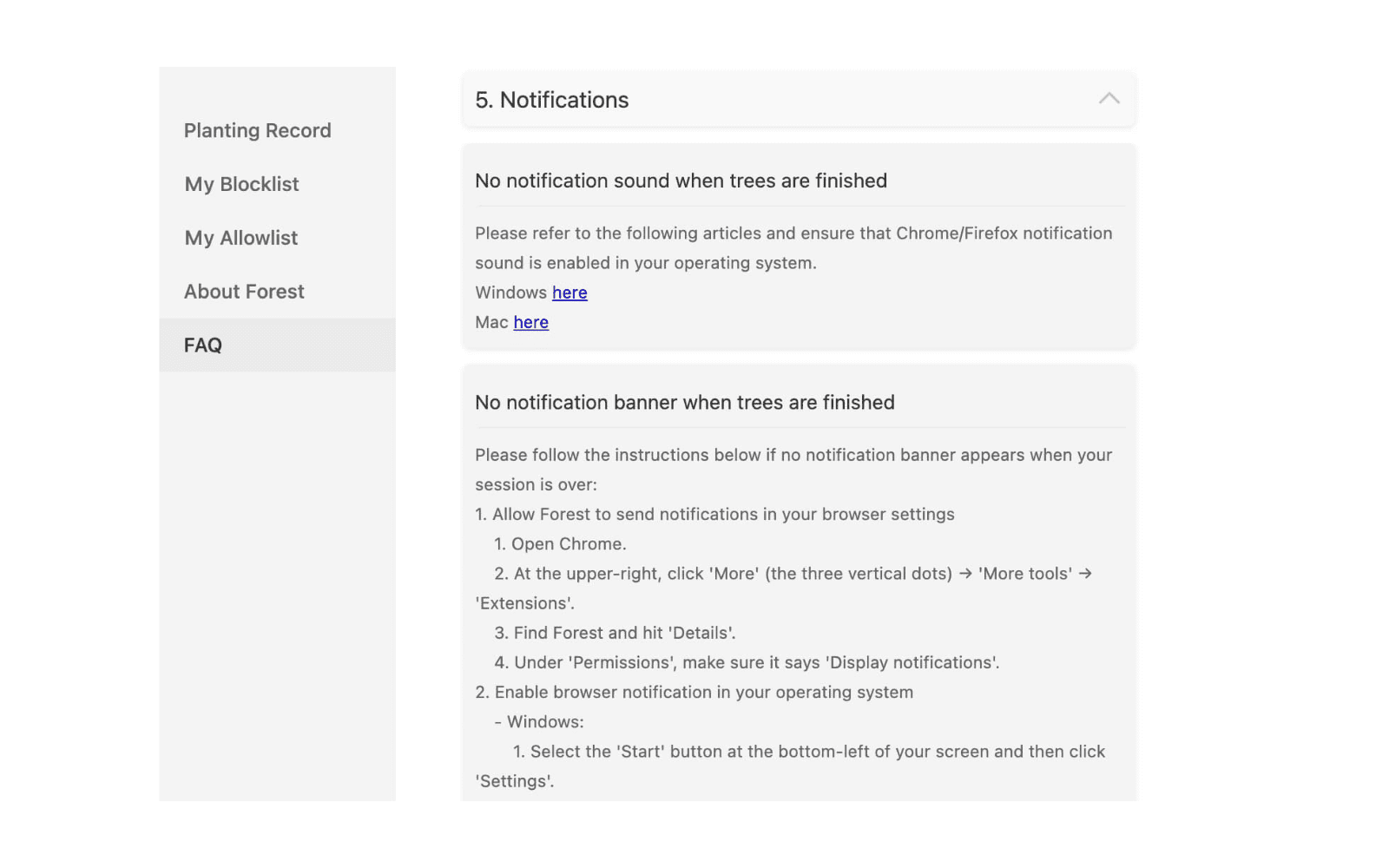The image features a gray background and displays a notification system with five pending notifications. Notably, there is no sound alert for the notifications. The image directs the viewer to refer to specific articles to enable Chrome or Firefox notification sounds on their operating system, with separate instructions for Windows and Mac outlined in blue text.

Additionally, there are troubleshooting steps in place for instances where no notification banner appears upon the completion of a task. The instructions provided include the following steps:

1. Allowing the app 'Forrest' to send notifications in your browser settings.
2. Opening Chrome and clicking on 'More' (three vertical dots) in the upper right corner, then navigating through 'Extensions,' finding 'Forrest,' clicking on 'Details,' and ensuring that under 'Permissions,' it is set to display notifications.

On the left side of the image, there is a menu featuring options such as 'Planting Record,' 'My Block List,' 'My Allow List,' 'About Forrest,' and 'FAQ,' with the 'FAQ' section highlighted in dark gray.

The text appears to end abruptly as the instructions are cut off.